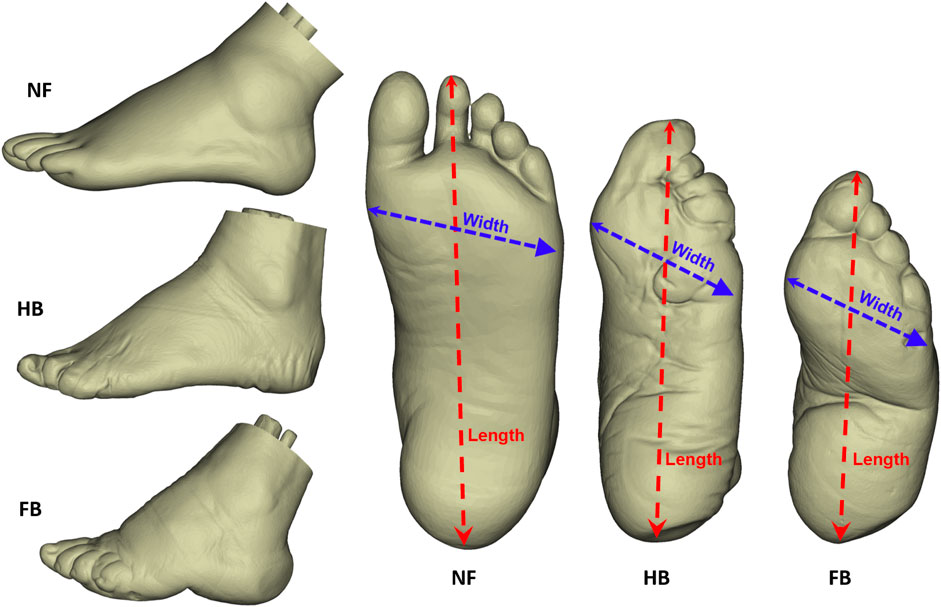This detailed illustration depicts six feet, split into two distinct columns. On the left-hand side, three feet are stacked vertically, presenting a side view. These feet are labeled as NF (normal foot), HB (half-bound foot), and FB (fully-bound foot), showing a progressive deformation. NF appears normal; HB shows initial signs of wrinkling and deformation; and FB is significantly scrunched and deformed, reflecting the stages of traditional foot binding. The feet are shaded brown and outlined in black. 

On the right-hand side, three feet are aligned horizontally in a row, each labeled similarly as NF, HB, and FB, displaying the bottom view. The first foot (NF) appears normal and is marked with a red dashed line labeled "length" from the big toe to the heel, and a blue diagonal line labeled "width" across the ball of the foot to the pinky toe. These notations illustrate measurements that change as the foot-binding process progresses. HB and FB follow, each increasingly scrunched and deformed, with their increasing wrinkling and curling of toes visually tracked by similar red and blue measurement lines. On the upper left of the image are the letters "NF," followed sequentially by "HB," and "FB" below each corresponding foot. These diagrams reflect the traditional Asian practice of foot binding, showcasing the physical transformations that occur over time.